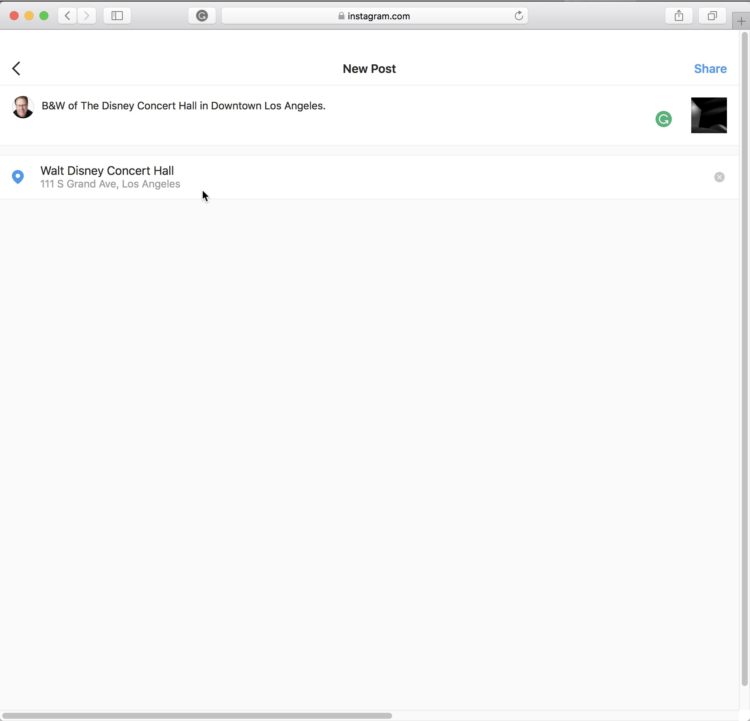The image depicts a social media post interface, presumably on Instagram. In the top right corner, there are three colored circles (red, orange, and yellow) representing window control buttons. Below them are navigation arrows—left and right—each in a separate white box, with an additional right arrow embedded within the latter. Adjacent to these, there's a small icon resembling a book.

Towards the center-right, there is a refresh button housed within a white box, next to a white rectangle displaying "Instagram.com." To its right, there is another, smaller refresh button. Farther right, an icon shows two overlapping squares, indicative of a gallery or layered photo setup, followed by an upload button.

In the lower section, the header reads "New Post" in the center, flanked by a left-pointing arrow to its left and a blue-highlighted "Share" button to its right. Below this, a profile picture is visible, accompanied by the caption "B&W of the Disney Concert Hall in downtown Los Angeles." Next to this caption on the right side is a green refresh button and a small, dark media image.

Further down, on the left side, there is a blue location icon labeled "Walt Disney Concert Hall," with the address "111 South Trot Avenue, Los Angeles" written in small print below. Finally, to the far right of this section, a small 'X' is present, likely for closing or discarding the post.